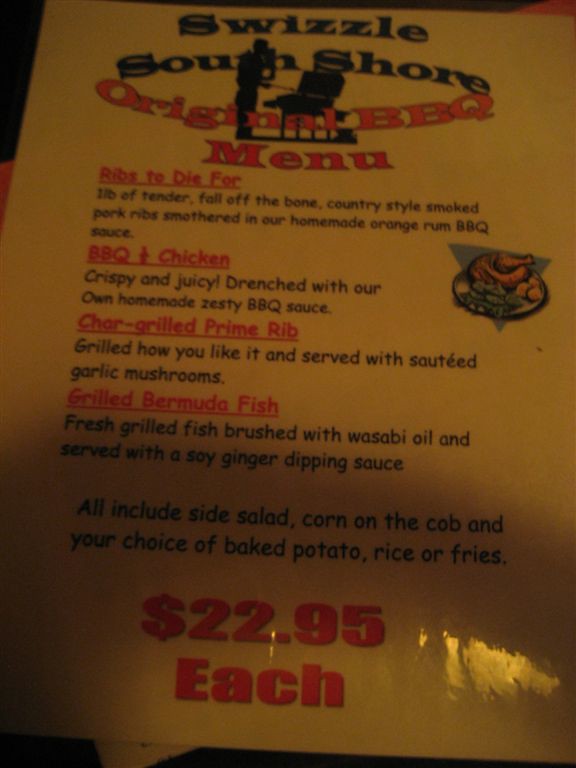This photograph captures a menu from Swizzle South Shore, though the image is quite dark and slightly blurry. The top part of the menu features a black header with the restaurant's name and an illustration of a person grilling on a barbecue. Below this, the menu is titled "Original Barbecue Menu". 

The first item is "Ribs to Die For" – described as one pound of tender, fall-off-the-bone, country-style smoked pork ribs, generously smothered in a homemade orange rum barbecue sauce. Following this is the "Barbecue Chicken," which is crispy, juicy, and drenched in a homemade zesty barbecue sauce. 

Next is "Char-Grilled Prime Rib," grilled to personal preference and served with sautéed garlic mushrooms. Another entree, "Grilled Bermuda Fish," features fresh fish brushed with wasabi oil and accompanied by a soy ginger dipping sauce. 

All meals come with a side salad, corn on the cob, and a choice of baked potato, rice, or fries. At the bottom of the menu, printed in red, is the price: $22.95 each.

Additionally, the top middle right of the photo shows what appears to be a plate of food, likely featuring chicken. In the bottom right corner, there is a small reflection of light.